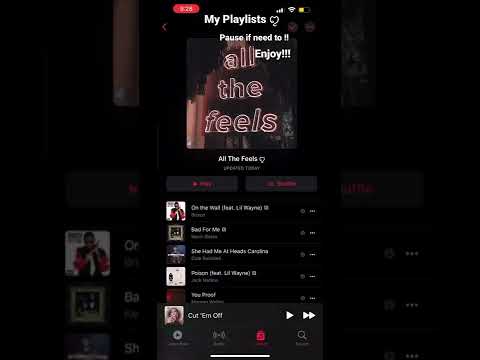The image is a vertically-oriented screenshot of an iPhone displaying the Apple Music app in night mode. The background of the image is a blurred, larger version of the same screenshot, adding depth to the scene.

At the top of the screenshot, typical phone status indicators are visible: the time on the left, and the signal strength, Wi-Fi, and battery icons on the right. Notably, the time is enclosed in a red rectangle, indicating that the screen is being recorded.

The Apple Music app is open to a section titled "My Playlist." At the top of this section, a user-caption reads "Pause if need to enjoy." Below this caption is the cover image of the playlist named "All the Feels," featuring an artistic blend of orange, red, and black hues.

The playlist title "All the Feels" is accompanied by a heart icon. Beneath the title are two buttons: one for play and another for shuffle. The body of the screen lists the songs in the playlist, each entry featuring a small image on the left, the song title on the top line, and the artist’s name below it.

At the bottom of the screen, a navigation bar offers additional options: Search, Library, Radio, and a display of what is currently playing.